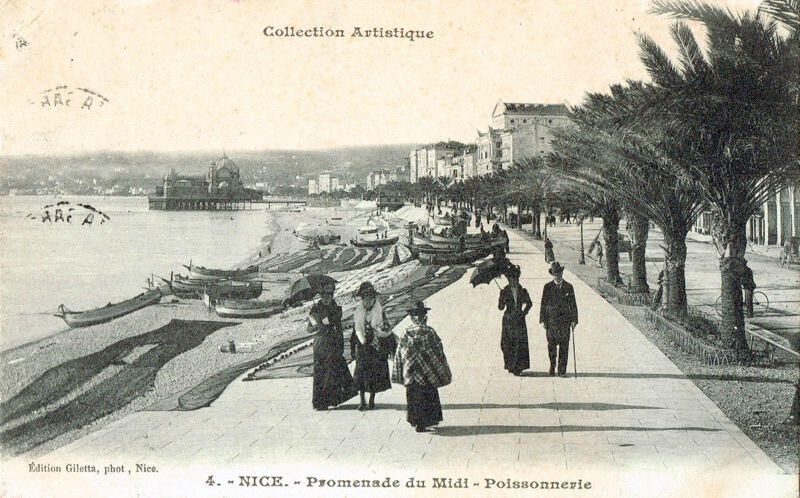This is a very old black-and-white photograph, possibly from the 1920s, labeled "Collection Artistique" at the top, and "Promenade du Midi" at the bottom. The image depicts a wealthy seaside area, likely in Italy, with well-dressed individuals strolling along a broad promenade. Women are seen wearing long skirts and holding umbrellas, while men don suits, ties, and top hats, one carrying a cane. The setting is a picturesque waterfront lined with palm trees on the right and water to the left, where beached gondolas lie adjacent to the promenade. In the distance, a dock and tall buildings come into view, emphasizing the affluence of the locale. The photo suggests a warm climate, capturing a serene and elegant atmosphere on a sunny day.